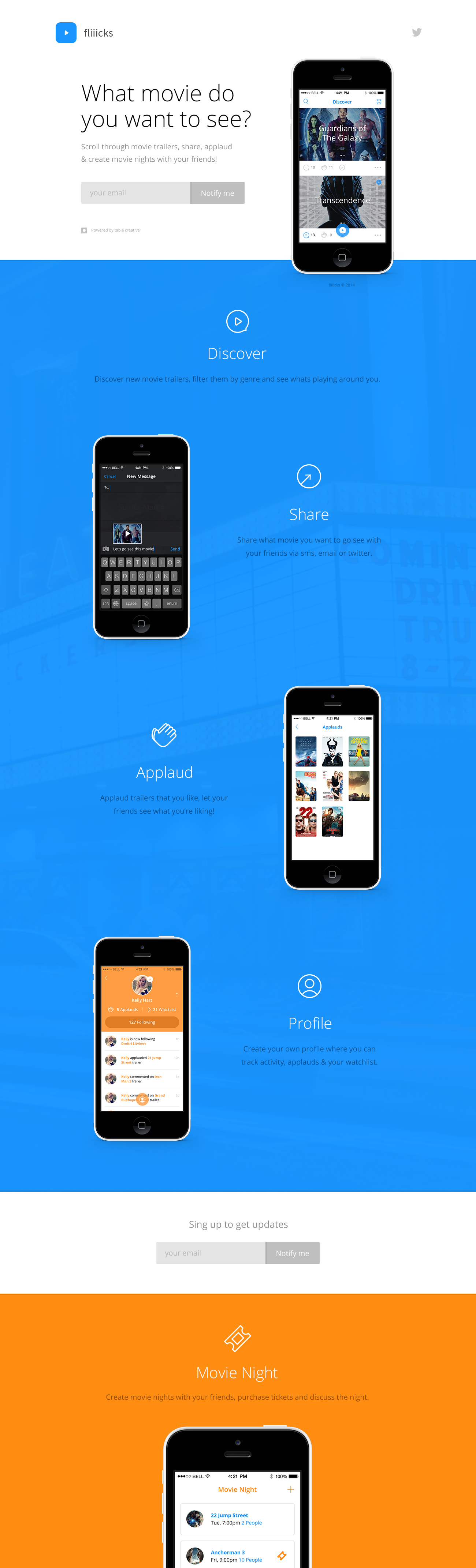The screenshot depicts the homepage of a website named "FLIIICKS". The header features a simple white background with a small blue rectangle containing a white right-facing carrot. On the far right corner, the gray Twitter bird icon is visible.

Below the header, a large text prompt asks, "What movie do you want to see?" followed by the suggestion to "Scroll through movie trailers, share, applaud, and create movie nights with your friends." This section includes a sign-up area with a gray bar for entering an email address and a button labeled "Notify Me" in a darker gray bar. The footer of this section mentions that the service is "Powered by TableCreative."

On the right side of the screen, there's a visual of a mobile device displaying apparent streaming content options for "Guardians of the Galaxy" and "Transcendence."

The background transitions to blue for the next section. In white text, it reads "Discover," accompanied by a bubble with a right-facing carrot. In darker text, the website explains: "Discover new movies, trailers, filter them by genre and see what's playing around you."

Moving right, a white circle with an upward-right arrow and the word "Share" below it introduces the sharing feature. In darker text, it elaborates: "Share what movie you want to go see with your friends via SMS, email, or Twitter." Adjacent to this text is an image of a cell phone displaying a movie picture and text message interface.

Further down, there's an icon of two white hands clapping with the word "Applaud" below. The caption explains: "Applaud trailers that you like, let your friends see what you're liking." To the right, another image of a mobile device shows movie options with an 'applaud' feature, presenting eight choices for applauding.

Leftward again, an illustration of a mobile device is seen next to a circle featuring a person icon, underlined with the word "Profile." The text invites users to "Create your own profile where you can track activity, applauds, and your watch list."

Following this, the background turns white. In gray text, it says "Sign up to get updates," with a gray bar for email entry and a "Notify Me" button.

The final section presents an orange background with a white outline of a movie ticket in the center, labeled "Movie Night" in white text. The accompanying darker text encourages users to "Create movie nights with your friends, purchase tickets, and discuss the night." Below this, another image showcases the top portion of a cell phone screen, which highlights the "Movie Night" feature with available movie options.

This detailed depiction of the "FLIIICKS" homepage effectively outlines its functionality, emphasizing movie discovery, trailer interaction, social sharing, and event planning.